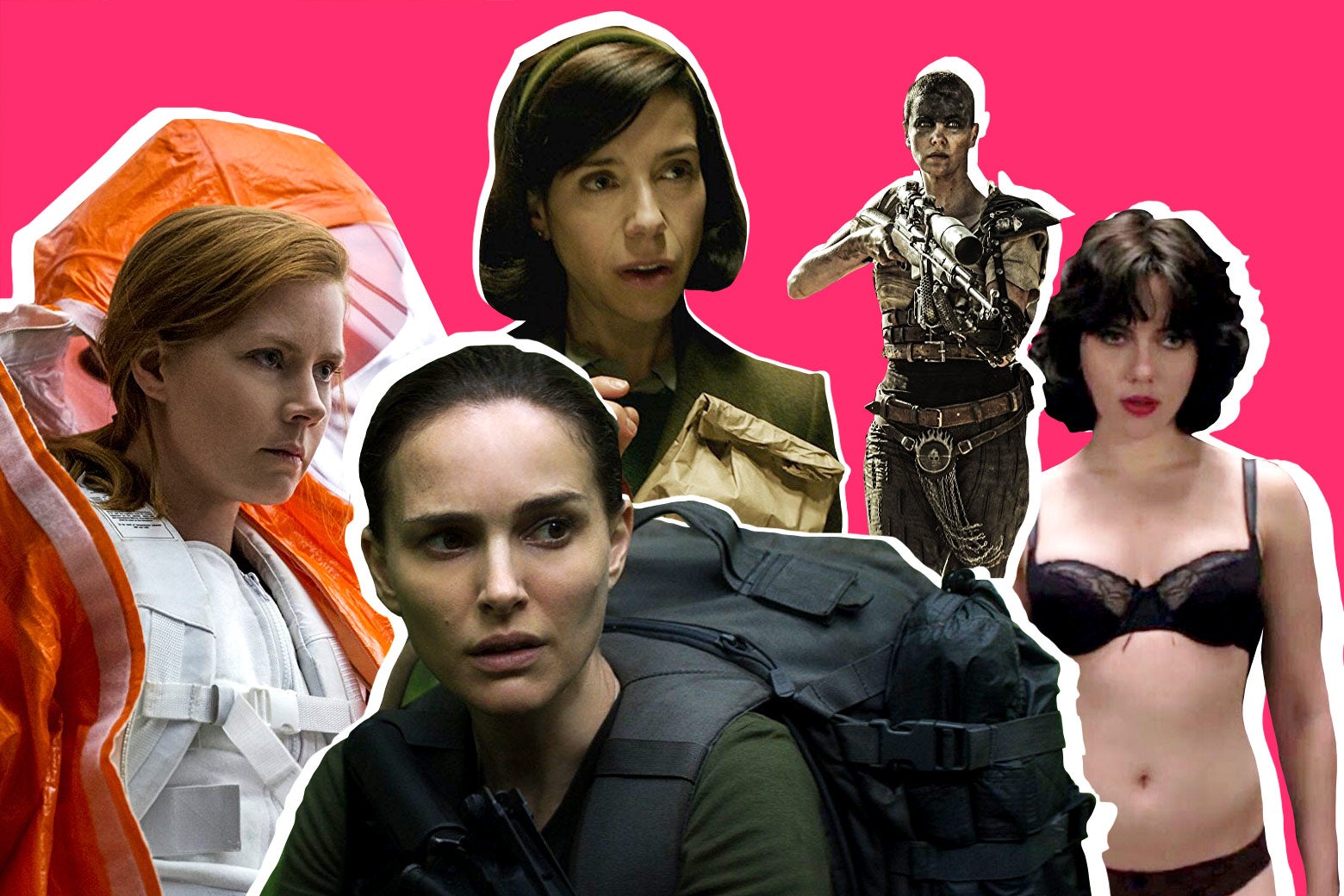This photoshopped collage showcases notable white actresses in their iconic film roles, set against a pink background. On the left is a red-haired woman in a white suit and orange jacket, possibly a character from "Outbreak." Below her is Natalie Portman from "Annihilation," with dark hair pulled back and equipped with a large black backpack. Above Portman, dressed in a 1940s-style army uniform and holding a paper bag, is a character likely from "The Shape of Water." In the center, Charlize Theron as Furiosa from "Mad Max: Fury Road" appears with a shaved head, makeshift armor, and a scoped gun. Finally, Scarlett Johansson from "Under the Skin" is on the far right, wearing only a bra and panties.